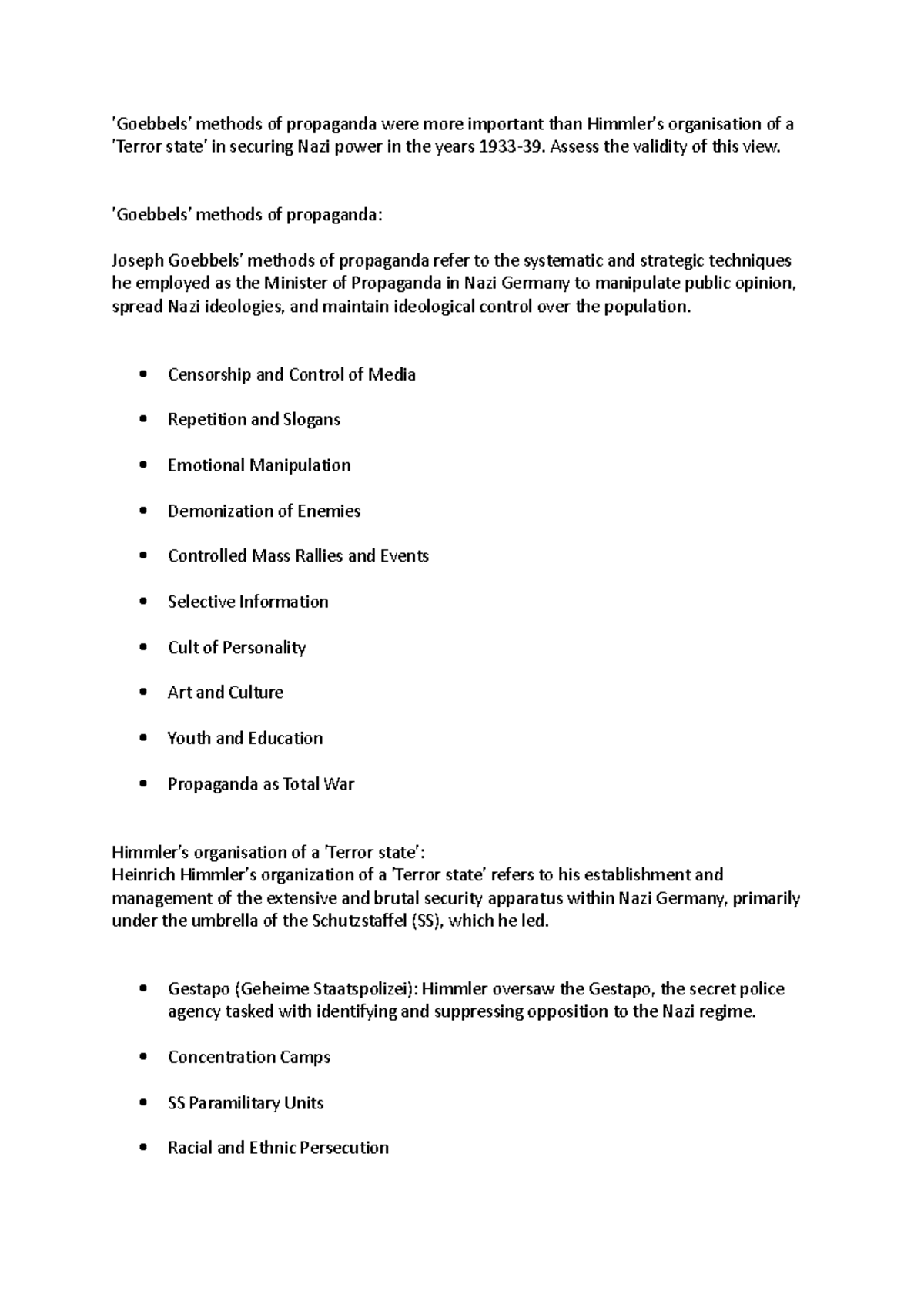The image depicts a screenshot from a digital text document with a white background. The text within the document is an assignment prompt for a historical analysis, reading: "Goebbels' methods of propaganda were more important than Himmler's organization of a terror state in securing Nazi power in the years 1933 to 39. Assess the validity of this view."

The document provides a detailed breakdown of the methods used by Joseph Goebbels and Heinrich Himmler to consolidate Nazi power from 1933 to 1939:

- **Goebbels’ Methods of Propaganda:** 
  - Joseph Goebbels, as the Minister of Propaganda, employed systematic and strategic techniques to manipulate public opinion, spread Nazi ideologies, and maintain ideological control over the population. 
  - The bullet points listed under his methods include:
    - Censorship and control of media
    - Repetition and slogans
    - Emotional manipulation
    - Demonization of enemies
    - Controlled mass rallies and events
    - Selective information
    - Cult of personality
    - Influence on art and culture
    - Impact on youth and education
    - The concept of propaganda as total war
  
- **Himmler’s Organization of a Terror State:** 
  - Heinrich Himmler’s role is described in terms of his establishment and management of the extensive and brutal security apparatus within Nazi Germany, primarily under the Schutzstaffel (SS), which he led.
  - His responsibilities included overseeing:
    - The Gestapo (Geheime Staatspolizei), the secret police agency tasked with identifying and suppressing opposition to the Nazi regime
    - Concentration camps
    - SS paramilitary units
    - Racial and ethnic persecution

This intricate comparison sets the stage for assessing the historical significance and relative impact of Goebbels' propaganda machinery versus Himmler's terror apparatus in the consolidation of Nazi power during the specified years.